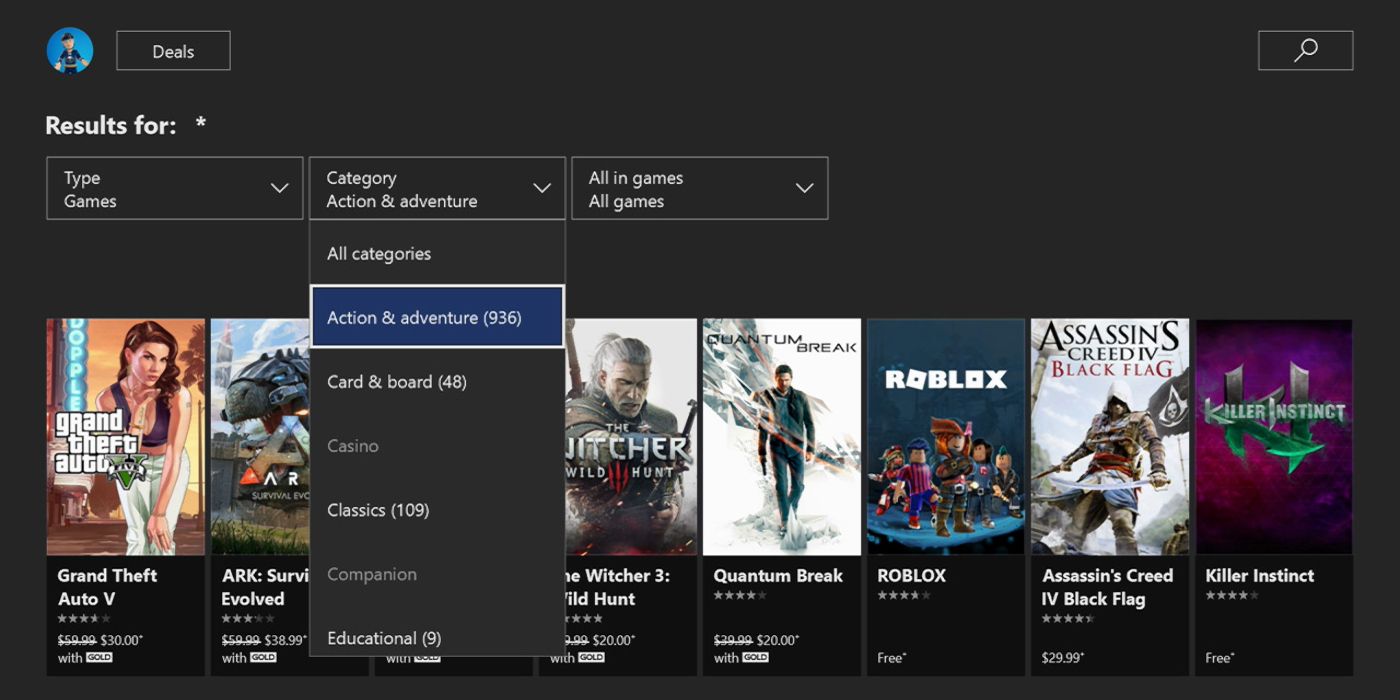The image depicts a landing page for a video game website. At the top left corner, there is a user icon featuring a cartoon female against a blue background. Adjacent to the user icon is a "Deals" button, which is styled in white text on a black background.

Below this header section, there is a results section that begins with the text "Results for" in white. This is followed by a series of drop-down boxes with white text on black backgrounds. The first drop-down box is labeled "Game Types." To its right, there is another drop-down box labeled "Category: Action and Adventure." Yet another drop-down box, labeled "All Games," is located further to the right. Beneath the "Category: Action and Adventure" box, the category is highlighted in blue, indicating it is currently selected.

Progressing downward, the page displays a selection of games with corresponding images. Starting from the left, the games listed are:
1. Grand Theft Auto V
2. Ark: Survival Evolved
3. The Witcher 3: Wild Hunt (positioned next to the drop-down box)
4. Quantum Break
5. Roblox
6. Assassin's Creed IV: Black Flag
7. Killer Instinct

Each game is represented by a distinct thumbnail image, making it easy for users to visually identify their choices.